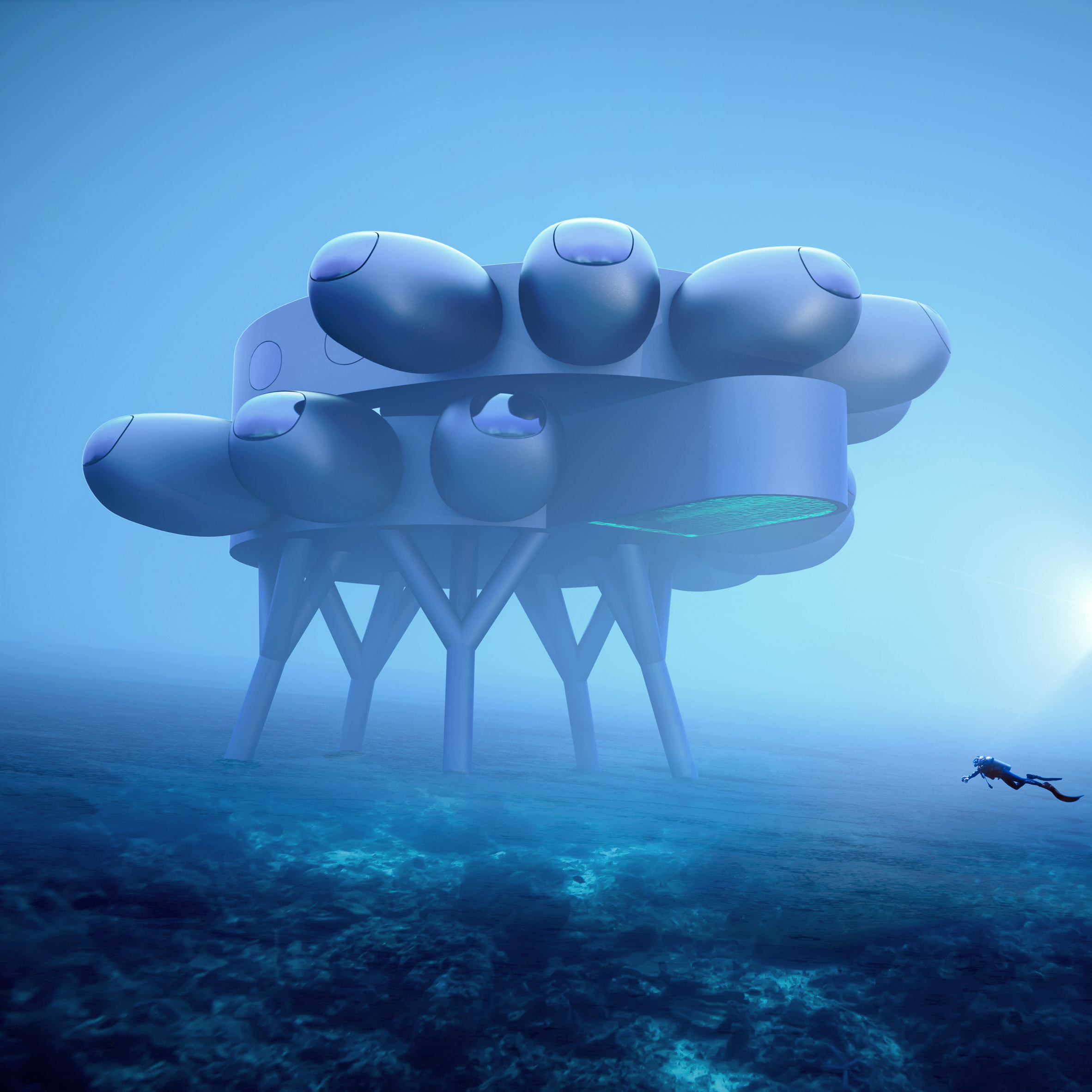An image depicts a highly detailed, possibly computer-generated scene set deep underwater. Dominated by hues of blue, the ocean floor appears to be a mix of coral and sandy terrain. Central to the image is a large, futuristic underwater structure, tinted in shades of purple. The structure is built on five sturdy legs and consists of two cylindrical sections stacked atop one another. Each cylinder features numerous pod-like extensions with windows, giving the impression of an advanced underwater residence or research station. To the right of the structure, a diver equipped with a scuba suit, oxygen tank, and flippers is seen approaching. The diver, though small in comparison to the immense structure, adds a sense of scale and realism to the scene. The background of the image fades into a deep blue, enhancing the mystery and depth of the underwater setting.